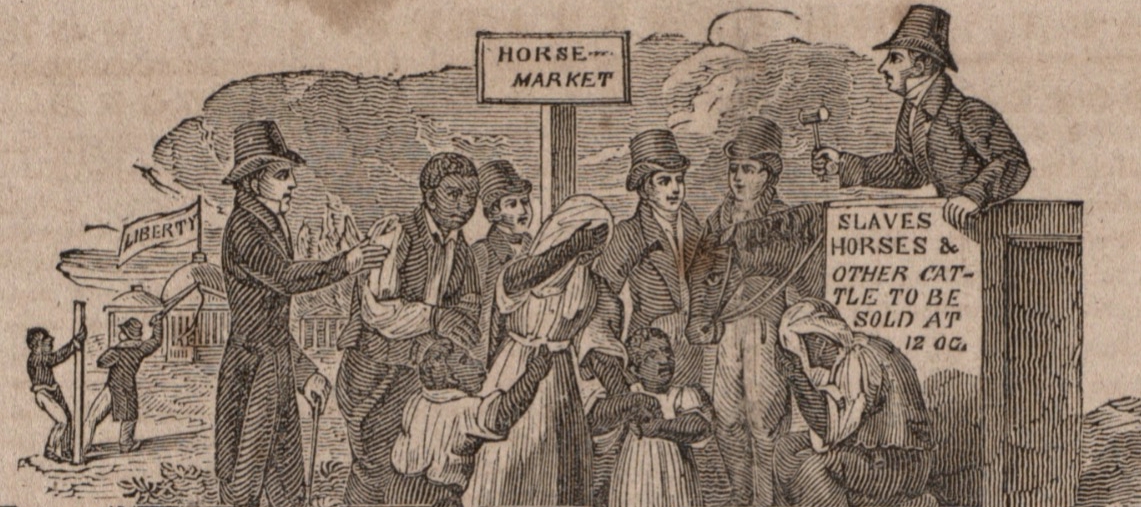The image is an old black-and-white drawing reminiscent of colonial-era political cartoons, printed on aged, grayish-brown paper. At the center, a sign reads "Horse Market," and nearby, a podium bears another sign stating "Slaves, horses, and other cattle to be sold at 12 o'clock." A white man in a suit and top hat stands at the podium, auctioneer's hammer in hand, orchestrating a slave auction. In the foreground, a distressed black family is depicted; the mother covers her face in sorrow as her two children cling to her sides. To the left, a white man is seen beating a black man who is tied to a pole. Surrounding the scene are white men in Victorian attire, illustrating the oppressive atmosphere. In the background, a building displays a flag with the word "Liberty," a stark contrast to the scene’s grim reality. Smoke rises from the buildings, and a horse stands near the podium. The image, dotted with intricate lines typical of prints from the 1860s, delivers a powerful anti-slavery message.